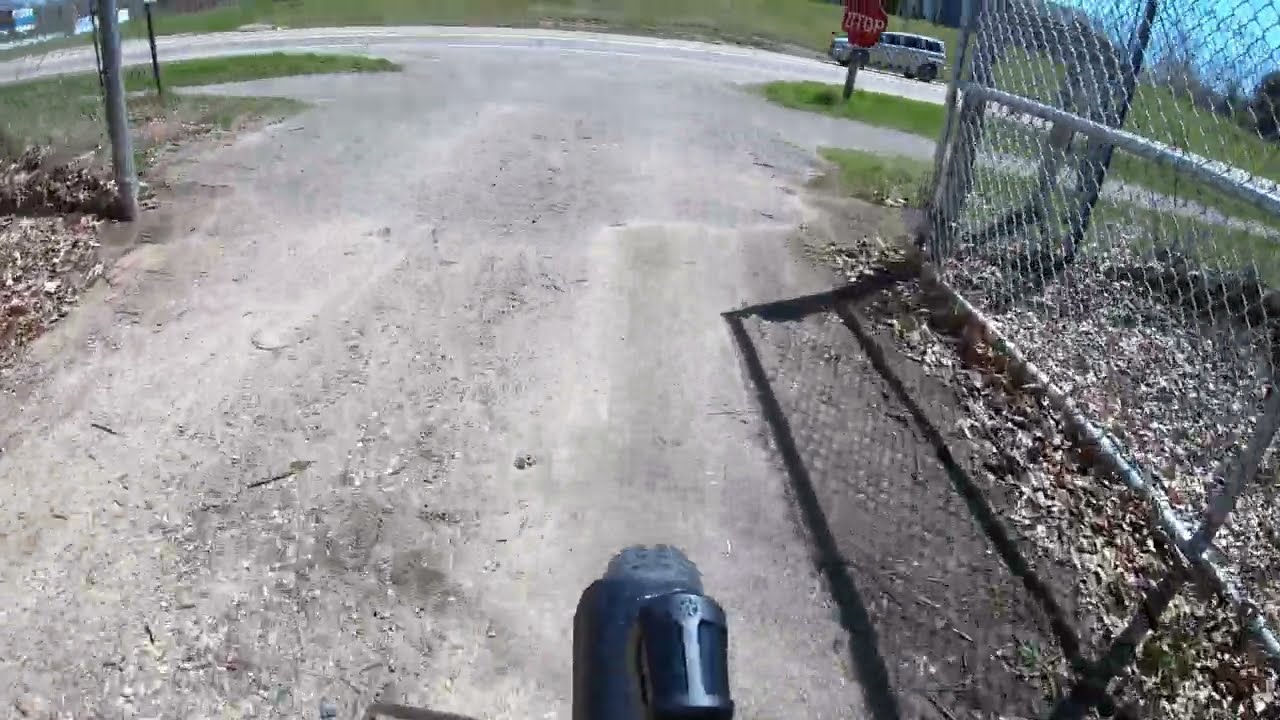The image captures an outdoor scene from the vantage point of an individual, possibly riding or walking, looking downwards at a dirt road. On the right side of this dirt road stands a tall chain-link fence, its shadow prominently cast onto the dirt surface. Dried leaves are scattered along the base of the fence and similar leaves litter the left side of the dirt road. 

At the end of the dirt road, a stop sign marks its intersection with a diagonal paved road in the background. A white sedan, which might be mistaken for a police vehicle, is parked on the opposite side of the paved road. Beyond the car, there lies a green, recently-mowed field under a clear blue sky. In the top right corner beyond the fence, a slightly blurred view reveals additional trees, indicating a rural or open-field setting on this sunny day.